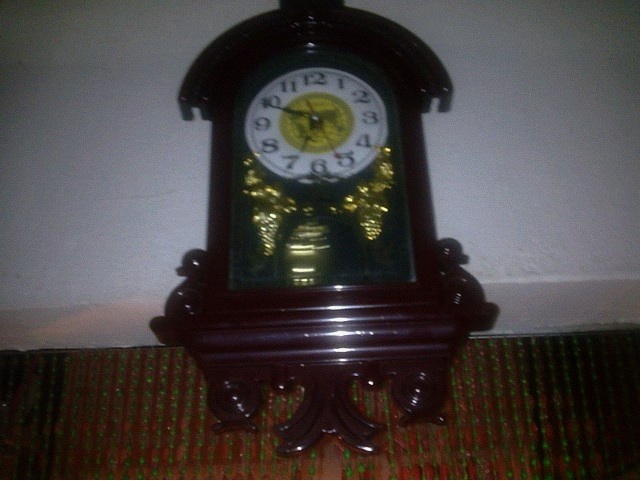In the image, there is a distinctive clock mounted on a red surface that appears to be made of either plastic or wood. The clock itself has a white, round face with clearly marked numbers from 1 to 12. At the center of the clock face is a prominent yellow circle. Surrounding the base of the clock are shiny gold objects positioned at the bottom left, right, and center, adding a decorative touch. 

The clock is resting on a red and green checkered mat, which adds a vibrant contrast to the scene. The background features a white, textured wall that appears bumpy, with a smooth base running along the bottom of the wall, providing a clean separation from the surface.

The clock's body has a unique shape, somewhat resembling an elongated form that widens and rounds out at the top, giving it a peculiar, almost whimsical appearance. At the base of the clock, on both the bottom left and right, there is a small, detailed duck figurine, adding a charming and playful element to the overall aesthetic of the setting.